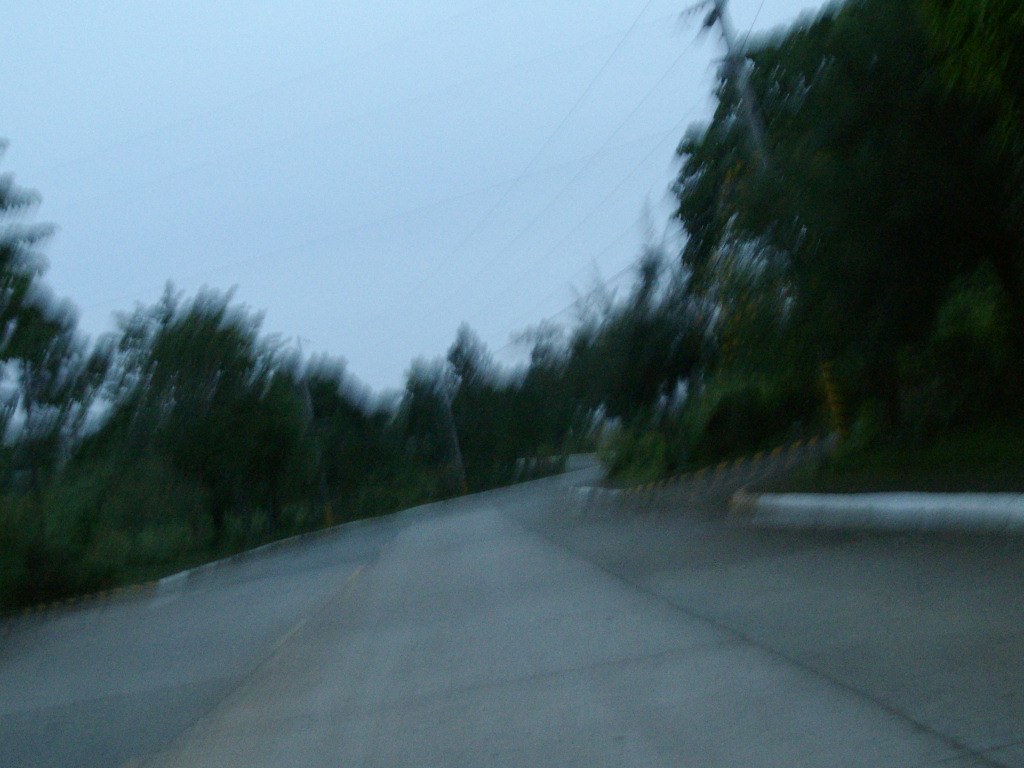This image appears to be taken from a dash cam or through the windshield of a vehicle traveling down a slightly wet, light gray asphalt road. The perspective is tilted, akin to the angle one might experience on a motorcycle about to make a turn. The road, which features a white dashed divider in the center, winds into the distance, curving right, then left, eventually disappearing into a dense line of fairly tall trees. Along the right-hand side, there is a white-painted curb and a driveway that ascends at an angle. Across from this, another junction branches off to the left. The scene is framed by tall telephone poles with connecting wires stretching across the road. The overall atmosphere suggests a muggy day, inferred from the lighting, but the sky remains clear and light blue. The photo, though blurry, captures the dense green foliage of grass, bushes, and trees lining both sides of the road, with a particularly full tree on the right and a taller tree on the left.